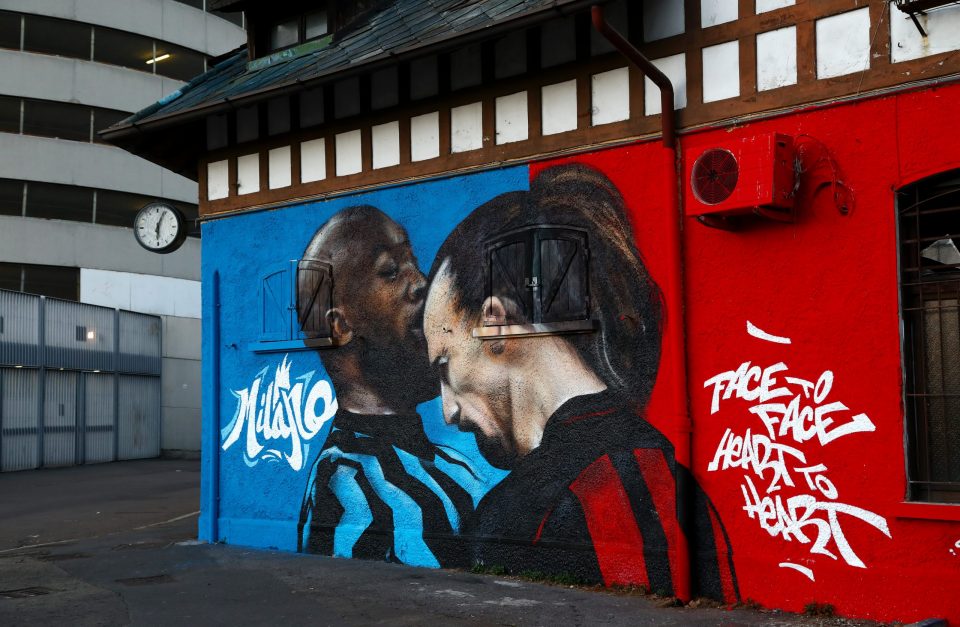This photograph features a vibrant mural on the side of a building, potentially located in Asia. The mural spans the entire wall and is distinctly divided into two colored sections: blue on the left and red on the right. Each side of the mural matches the clothes worn by the two depicted individuals. 

On the blue side, there is a dark-skinned man wearing a blue and black striped shirt, with the graffiti text "Malaro" (potentially "Milano") positioned beside him. He is gently kissing the forehead of the man on the right. The right side of the mural shows a light-skinned man with long black hair in a ponytail, wearing a red and black striped shirt. His head is tilted down with eyes closed, and he sports a goatee. Beside him, the graffiti reads "face-to-face, heart-to-heart," in bold white text, framed by thin lines above and below the text.

To the left of the mural-colored building, there is a white building with a clock mounted at the top, showing the time as 6:05. The ground in front of these structures is dark gray in color.